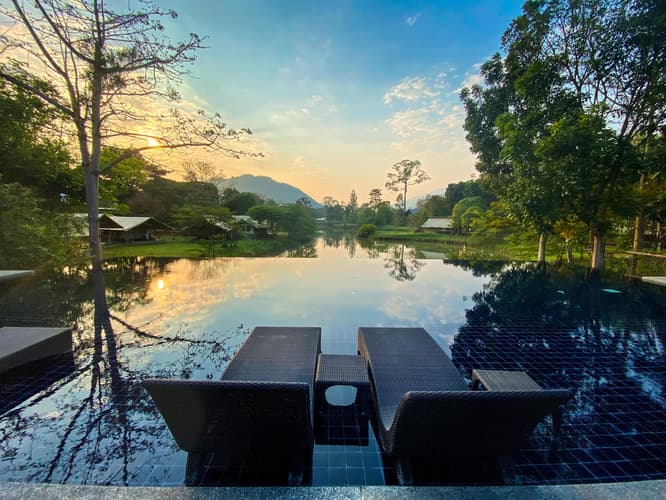This serene sunset photograph captures an opulent outdoor scene featuring an exquisite infinity swimming pool with a backdrop that seamlessly blends into nature. In the foreground, two reclining pool chairs are partially submerged in about a foot of water, providing a unique in-pool lounging experience. A small table between the chairs offers a convenient spot for drinks or reading materials. The pool's interior is adorned with dark blue tiles, adding to the luxurious feel. The pool appears edgeless, extending into a reflective body of water that merges beautifully into a lush landscape filled with verdant grass and trees. Farther out, a river or waterway creates a picturesque bayou-like setting, with a couple of houses nestled amidst the greenery. The sky is mostly clear, painted with a golden glow from the setting sun on the left, casting a tranquil ambiance. The mountains in the distant background complete this captivating and tranquil scene, making it a perfect escape into nature's beauty.